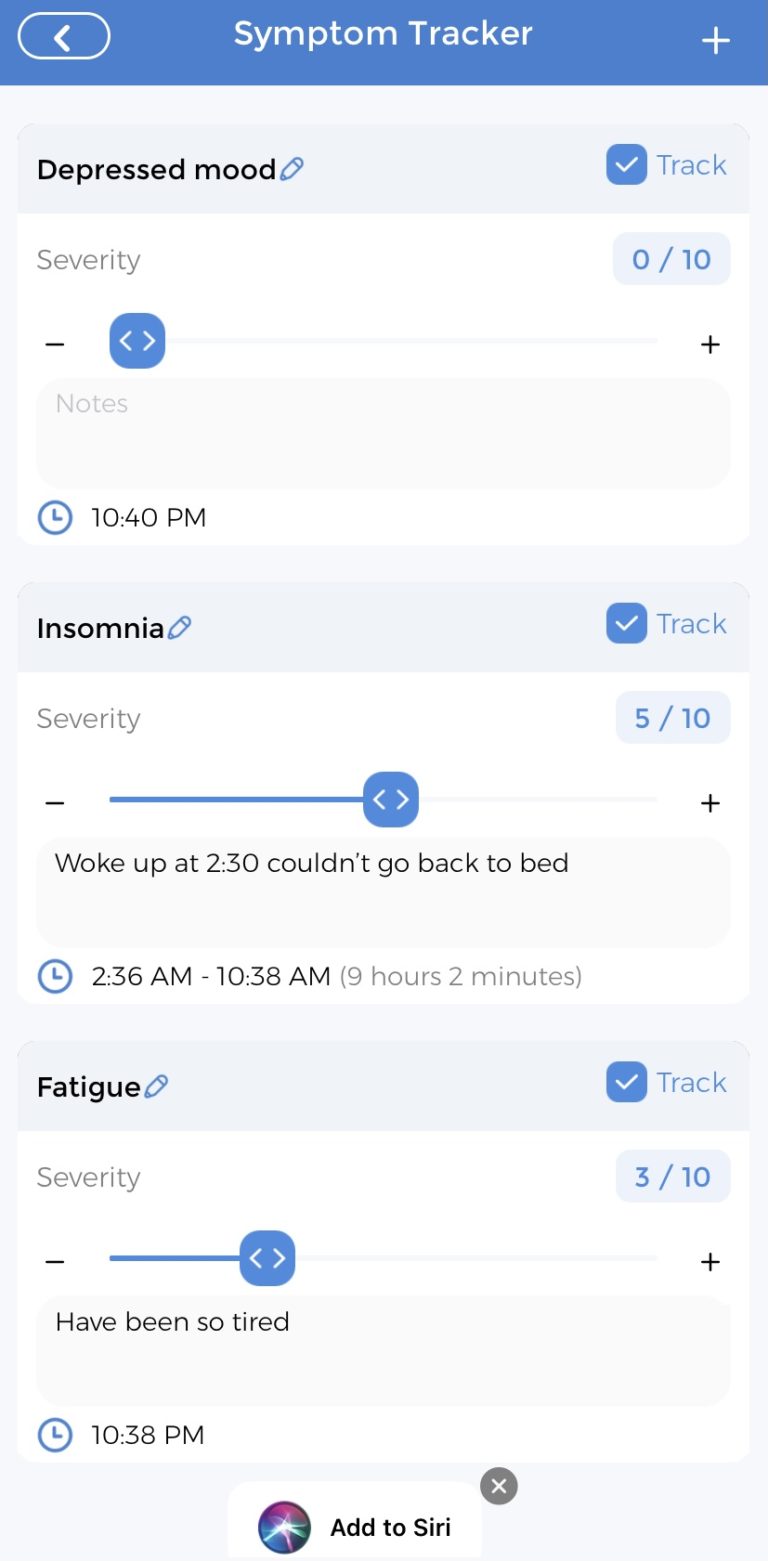The image displays a highly interactive telehealth program interface focused on tracking symptoms. The page prominently features a 'Symptom Tracker' section with a circular arrow to the left and a plus sign to the right, all set against a blue background. 

The first symptom listed is 'Depressed Mood,' accompanied by a crayon icon for notes and a checkmark indicating it is being tracked. Users are prompted to rate the severity of their mood on a scale from 0 to 10 and can add additional notes. The page includes a timestamp noting an entry made at 10:40 p.m.

Below this, the symptom of 'Insomnia' is detailed. A similar crayon icon and checkmark are present. The severity of insomnia is marked as 5 out of 10. A note beside it states, "Woke up at 2:30, couldn't go back to bed," with tracked sleep duration from 2:36 a.m. to 10:38 a.m., totaling 9 hours and 2 minutes of sleep.

The third symptom, 'Fatigue,' is also included with an associated crayon icon and a checkmark for tracking. It is rated at a severity of 3 out of 10, with a note saying, "Have been so tired," recorded at 10:38 p.m. 

The interface offers options to integrate the symptoms with 'Siri' or to exit the tracker.